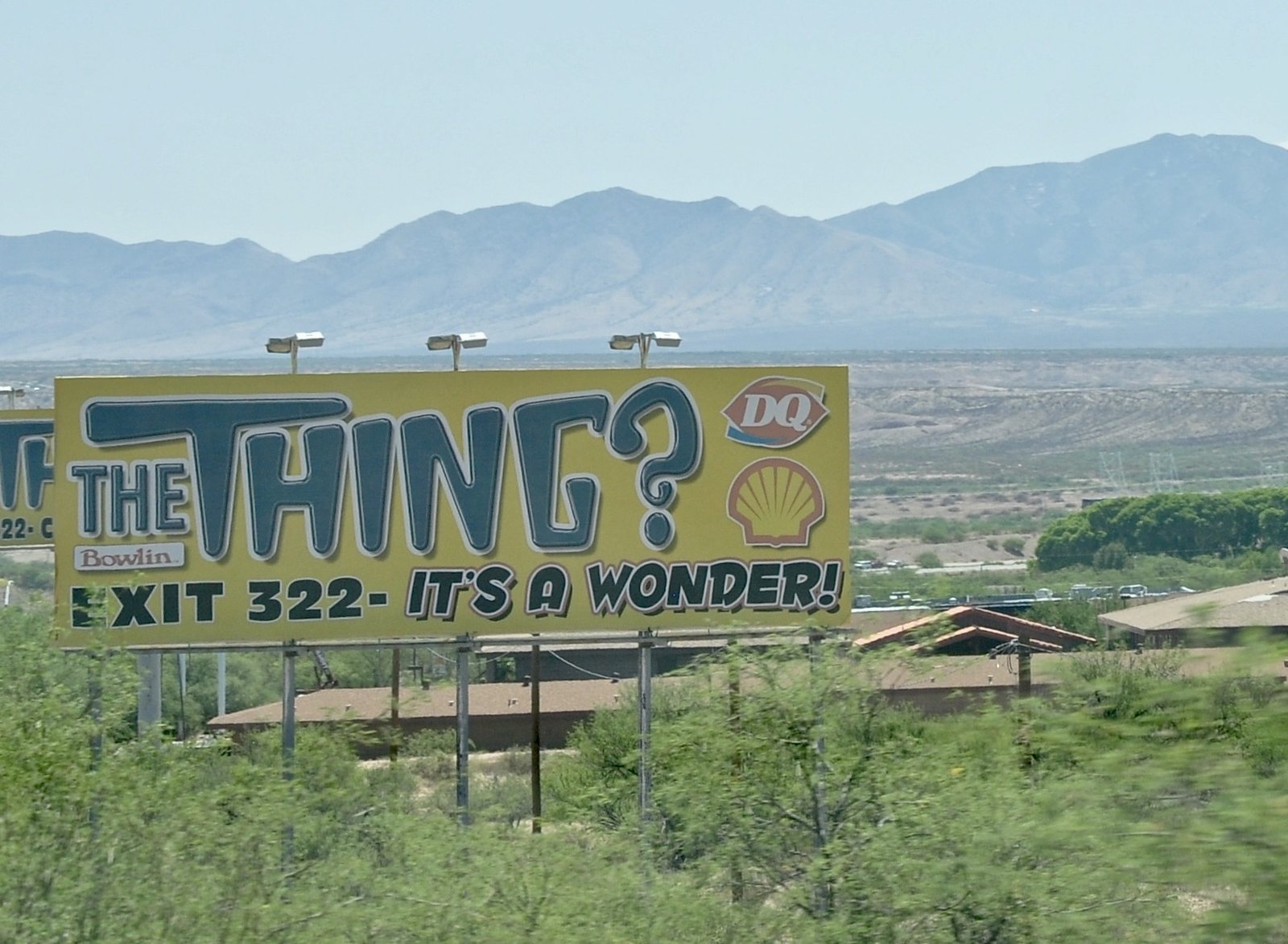This photograph captures a rural, desert-like landscape seen from a moving vehicle on a highway. The image, dominated by a vast expanse of dry, flat land with scattered, scrubby brush and low-lying trees, unfolds in the foreground. Some of these trees have a slight motion blur, evidencing that the photo was taken from a moving car. In the middle ground, there are rooftops of houses partially obscured by the sparse foliage. The backdrop features a range of brown mountains under a hazy, whitish-blue sky.

The most striking element is a prominent yellow billboard towering above the scene. Two identical billboards are visible, one stacked behind the other. The billboard, featuring bold black text, poses the intriguing question, "The Thing?" and in smaller text below, the name "Bolin." To the right, the ad includes symbols for Dairy Queen and Shell gas station, positioned above the directive, "Exit 322," followed by the exclamation, "It's a wonder!"